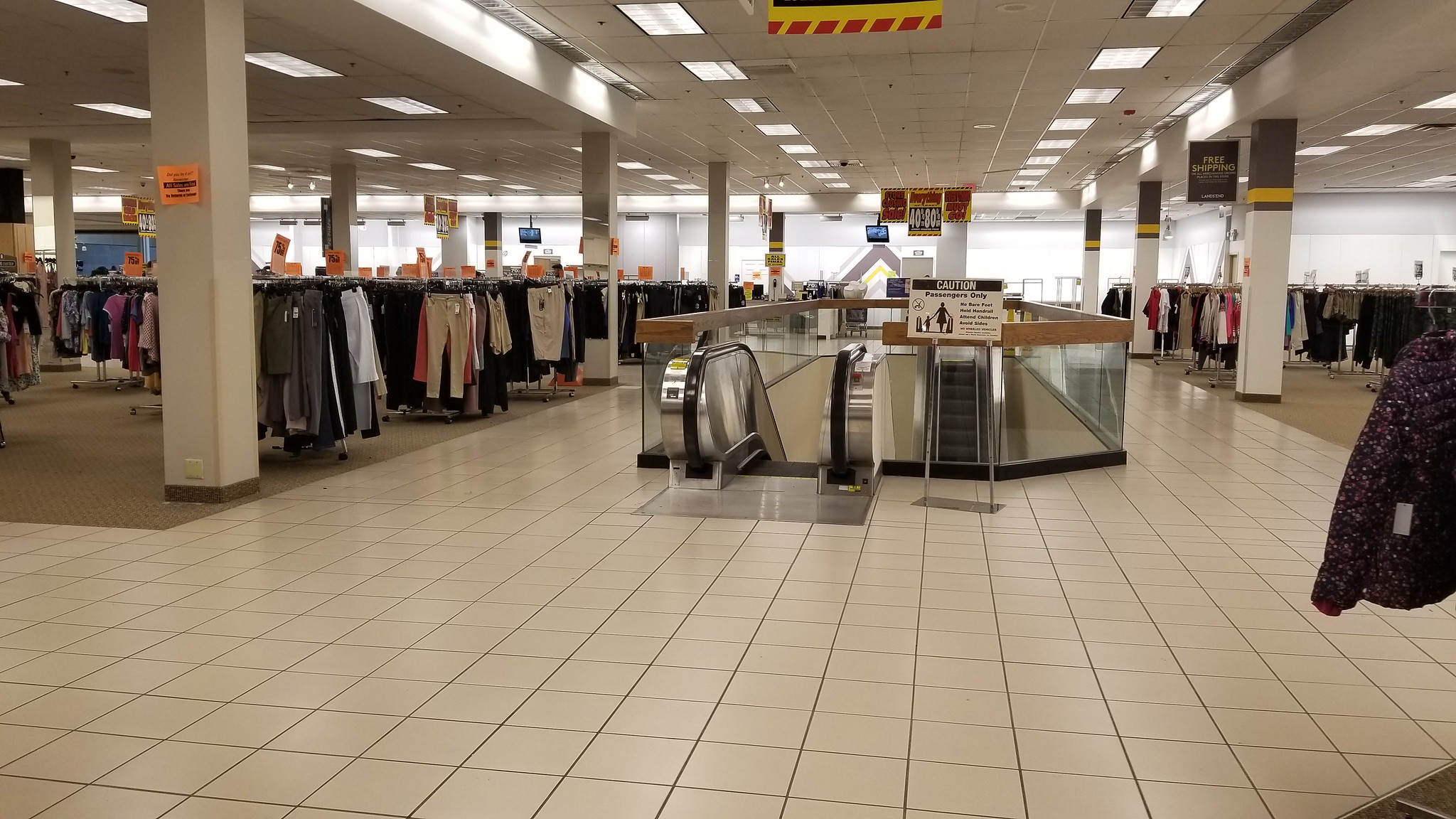This photograph captures the interior of a department store reminiscent of J.C. Penney or Sears. The left side of the image is filled with an array of clothes, prominently featuring pants. The right side showcases shirts, blazers, and long-sleeved coats neatly arranged. Positioned centrally are two escalators - one descending and the other ascending to an upper level. The store is notably clean, with the walls painted a warm tan color. The flooring in the main walkways consists of tan-colored tiles, complemented by darker brown-gray carpeting flanking the sides. The silver escalators stand out, and a caution or warning sign is visible nearby, emphasizing safety. The overall ambiance exudes a welcoming and organized shopping environment.